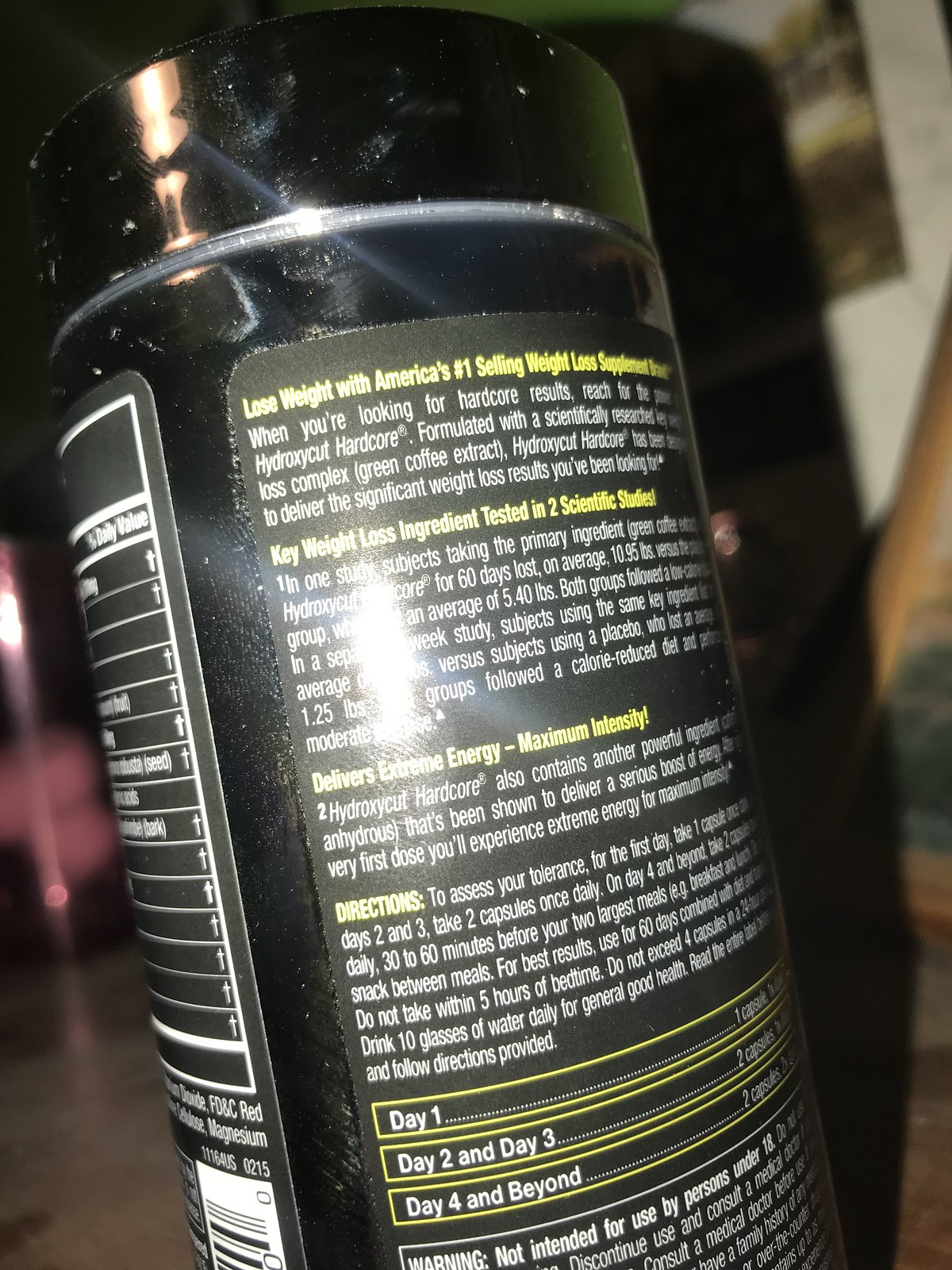This photograph features a bottle of a weight loss supplement, prominently showcasing a bronze-colored cap. The bottle itself appears to be made of either glass or plastic, reflecting light off its label, particularly towards the middle and upper parts. The label proclaims this product as America's number one selling weight loss supplement, designed for those seeking hardcore results. It emphasizes the inclusion of a scientifically researched weight loss complex with green coffee extract. The brand, Hydroxycut Hardcore, promises significant weight loss outcomes.

The label, predominantly black with white and yellow text, contains extensive information, including directions for use and a warning label at the bottom. Some text on the right-hand side of the label is obscured and unreadable. The partial view of the nutrition label is visible on the left side, due to the angle at which the bottle is positioned. In the background, there is some shadowing, and an out-of-focus vision reveals an off-white wall adorned with a picture. There also appears to be a staircase or a chair towards the right side of the image.